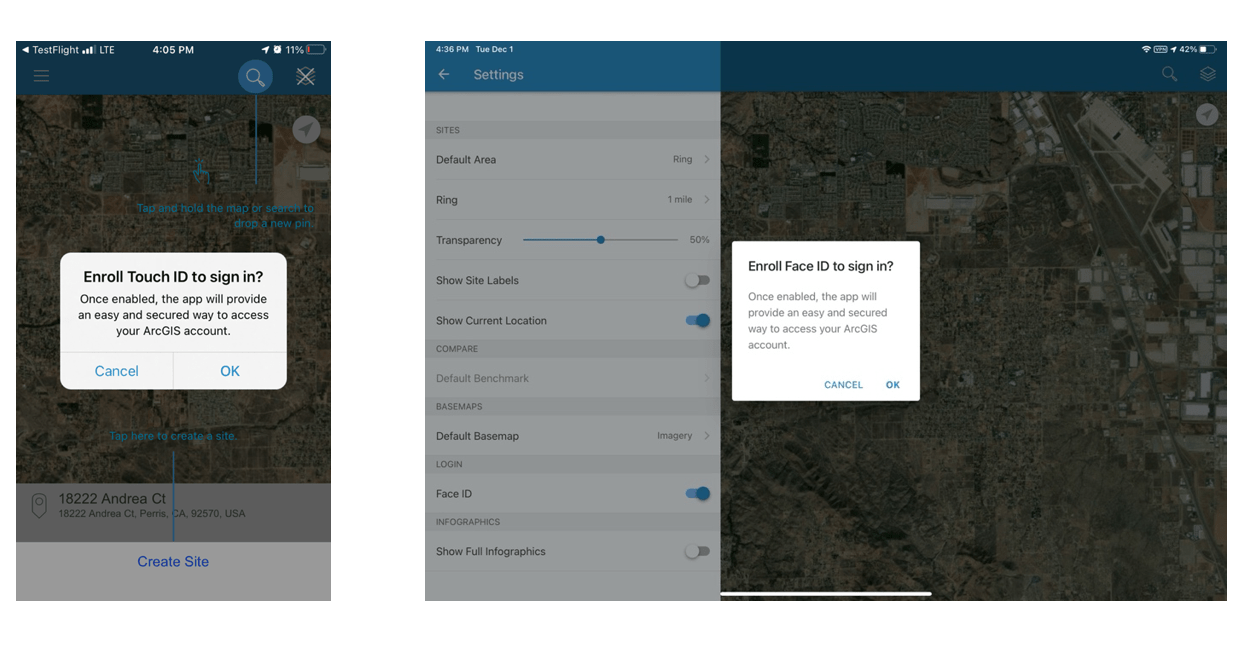**Detailed Caption:**

The image is a set of two screenshots showcasing different devices accessing the ARCGIS application. 

The screenshot on the left is from a cell phone display. At the top of the screen, it shows the notification bar with the label "Test Flight LTE", along with the time, indicated as 4 or 5 p.m., and the battery level at 11%. The main section of the screen features a dark map overlaid with blue text that instructs users to "Tap and hold the map or search to drop a new pin." In the foreground, there's a prominent white popup window displaying a message that reads, "Enroll Touch ID to sign in. Once enabled the app will provide an easy and secure way to access your ARCGIS account." There are two options at the bottom of this popup: "Cancel" and "OK." At the bottom of the screen, another instruction reads, "Tap here to create a site," with a blue line pointing downwards towards the same label. Additionally, the address 18222 Andrea Court, Perris, California 92570 USA, is visible on this screen.

The screenshot on the right is from a computer interface. The far left of the screen features a greyed-out menu with various settings options, including "Default area ring: 1 mile," "Transparency: 50%," "Show site labels," "Show current location on compare," "Default benchmark," "Default base map," "Face ID on," and "Show full infographics." The background also consists of a very dark map. In this screenshot, a similar white popup window appears, with the message, "Enroll Face ID to sign in. Once enabled the app will provide an easy and secure way to access your ARCGIS account." This popup also includes the options "Cancel" and "OK."

Both screenshots highlight the security features for signing into the ARCGIS application, one using Touch ID on a mobile device and the other using Face ID on a computer.